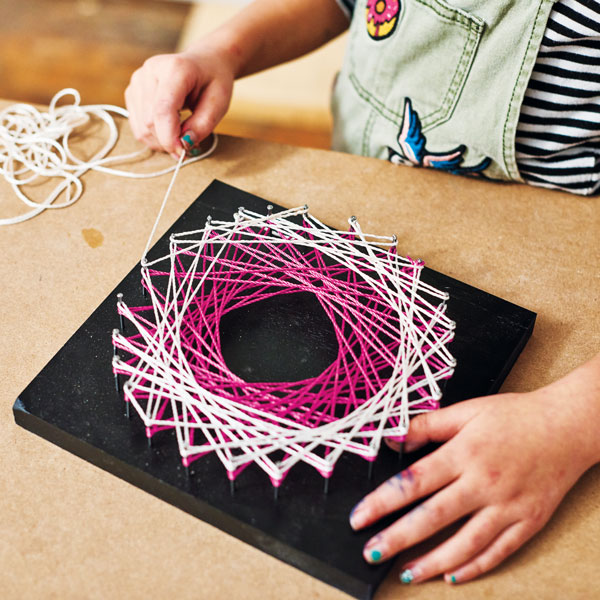A person, whose gender is difficult to determine, is photographed at a wooden table, engaged in crafting a string art project. The image only reveals their torso, chest, left arm, and hand. They are dressed in faded blue jean overalls adorned with patches—one depicting a pink donut trimmed in yellow, and the other showing a partial blue bird—and a navy and white striped shirt. Their left hand, smeared with blue, pink, and yellow paint, is working with pink and white threads on a black square wooden board. The threads are woven into a circular pattern. The person appears to have scratched-off blue nail polish on their fingers, adding to the creative and colorful scene.